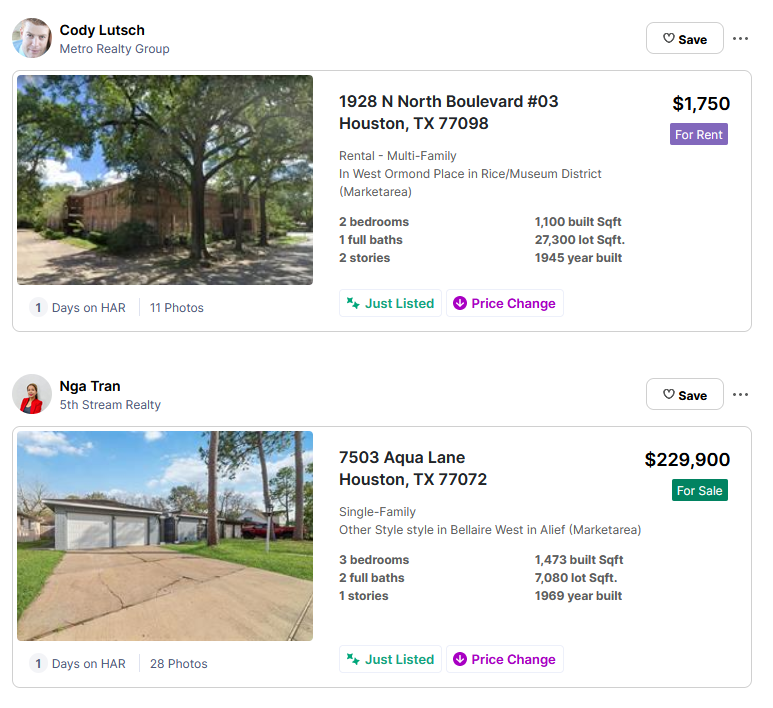Here is a polished and detailed caption for the image:

---

This photograph showcases two properties, both situated in Houston, Texas, and listed by Cody Lutsch of Metro Realty Group. On the left is a rental property listed for $1,750 per month. This charming two-bedroom, one-bath home is spread across two stories and boasts a retro appeal, having been built in 1945. The rental property is located on North Boulevard and encompasses approximately 1,100 square feet.

On the right is a single-family house available for sale at $229,900. This property offers three bedrooms and two bathrooms, all on a single story. Constructed in 1969, this home spans 1,473 square feet and is situated on Aqua Lane. Both homes exude a distinct architectural charm and are nestled within the vibrant community of Houston.

---